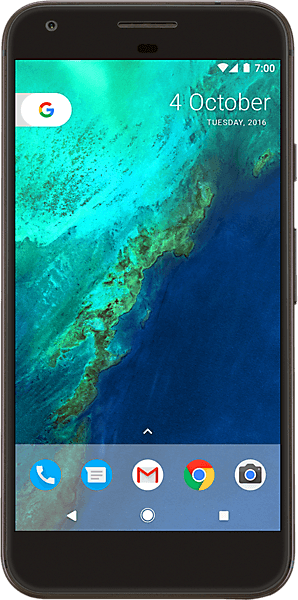A high-resolution image depicts a black Android smartphone, easily identifiable by the navigation icons at the bottom—a back arrow, a circle, and a square. On the right side of the device, three buttons are visible: one smaller button positioned above two slightly larger ones. At the top-right corner, there is a pinhole likely for a secondary microphone or camera, accompanied by a rectangular slot serving as the speaker and volume control.

The phone's screen shows a vivid tropical ocean scene, possibly a beach or island, as its wallpaper. The status bar at the top reveals full Wi-Fi signal, full cellular signal, and a fully charged battery, alongside the time, 7 a.m., and date, Tuesday, October 4th, 2016. The top-left corner features a Google 'G' logo, indicating a quick access option for Google search.

At the bottom of the screen, a small upward-pointing arrow suggests expandable or collapsible options. The dock includes several app icons: a blue circle with a white headset symbol for calls, a blue circle with a white chat bubble for text messages, a white circle with a red outlined envelope for email, the Google Chrome icon featuring a blue circle with a tri-colored ring in red, yellow, and green, and a camera icon designed with a classic camera illustration and a blue lens.

This image offers a detailed view of a typical Android smartphone interface from 2016, showcasing its physical design and on-screen elements.